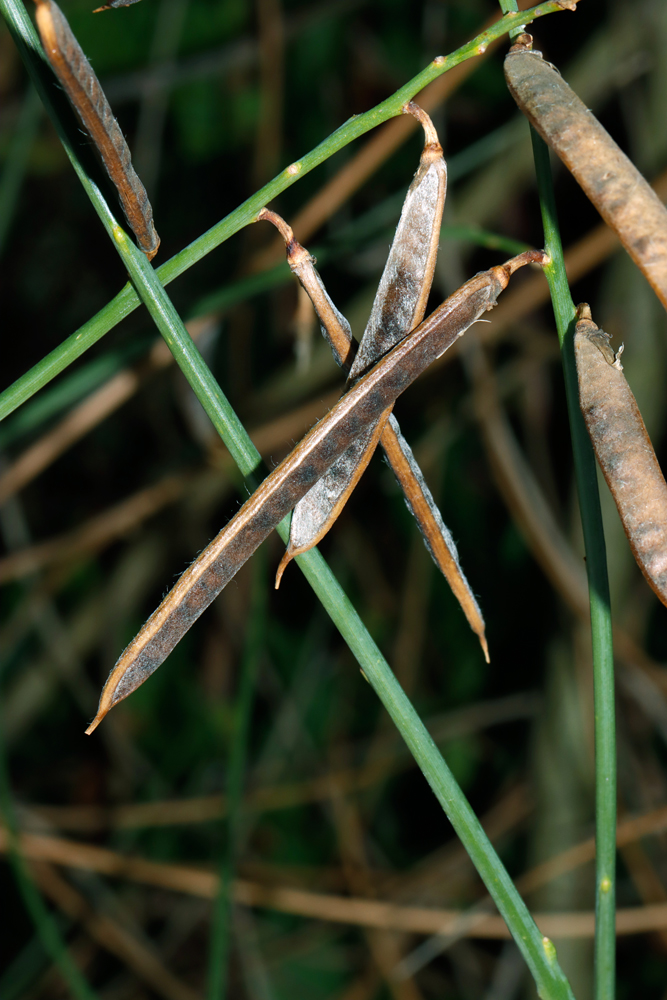The high-resolution photograph captures a close-up view of a leguminous plant with slender green stems, devoid of leaves, showcasing clusters of dried, elongated brown seed pods resembling flat string beans. The vivid green stems contrast with the brown pods, hinting that parts of the plant are still verdant while others have died. Intermixed with these stems are likely long, slender blades of grass, adding to the greenery. In the blurred background, other grasses can be seen, emphasizing the plant’s natural environment. The seed pods, attached to the green stalks, hang downward, indicating the late stage of the plant’s life cycle where the leaves have already fallen. This nature shot provides a detailed study of the plant’s anatomy amidst a serene, slightly out-of-focus backdrop, most likely in a natural or forest-like setting.